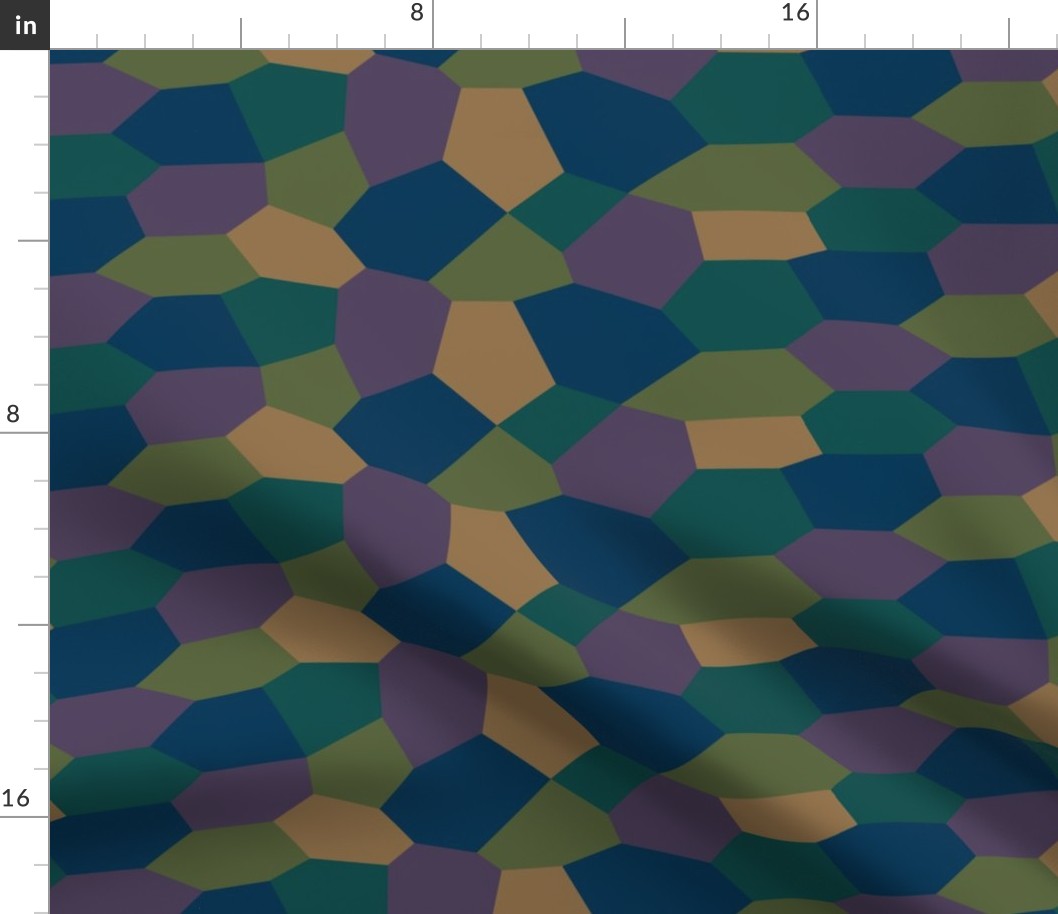The image showcases a tessellating pattern resembling an Escher print or a quilt, with a variety of geometric shapes combining to form a complex design. Featuring around a dozen different shapes, the pattern includes shapes predominantly with five or six sides, though there are also occasional four-sided and varied-sized shapes. The colors used are a rich palette of blue, light green, darker green, beige, purple, navy, teal, lime green, and yellowish tan. Some patches give an impression of fabric with a wavy effect, particularly noticeable in the bottom third of the image. 

The overall design appears on a purple background, with measurement scales visible along the sides in inches. The top and bottom scales extend beyond 16 inches, with the left-hand side reaching up to 18 inches and the right-hand side extending to 21 inches. Additional measurement markings displaying numbers 8 and 16 are prominently featured in black text arranged along the top and left edges, adding a precise, grid-like structure to the visual complexity of the pattern.